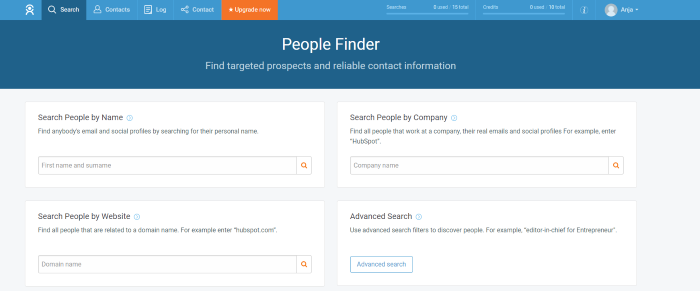Screenshot of People Finder website's main page.

The top portion of the page is adorned with varying shades of blue, contrasted by a small orange rectangle offering an option to upgrade the system, accessible at any time with a simple click. The remainder of the page features white text instructions formatted as drop-down menus, allowing users to navigate different parts of the site.

A small thumbnail icon confirms that the user is signed into their account. Below this section, a prominent banner reads "People Finder" along with the tagline "Find targeted prospects and reliable contact information."

The background shifts to white as users scroll down further, revealing four sizable rectangles, each equipped with a search box. Each rectangle has bolded blue text describing different search functionalities:
1. Search by Name
2. Search People by Company
3. Search by Different Websites
4. Advanced Search

The advanced search option includes a secondary menu for additional search parameters.